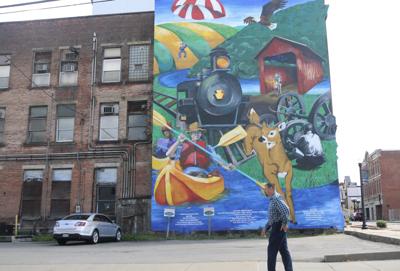In this vibrant city scene, a man dressed in dark blue walks along a sidewalk, centrally positioned in the image, with the striking backdrop of a large, colorful mural painted on the side of a red brick apartment building. The mural is an elaborate, vivid depiction featuring various elements: at the bottom, two people are kayaking in yellow boats on blue water, while a deer leaps into the scene. Above them, a black steam locomotive rides along railroad tracks. To the right, a farmer plows a field, and behind him, a red barn can be seen against green hills. Higher up, a man parachutes down from the sky. The mural boasts a spectrum of bold colors including green, red, black, orange, and yellow. Adjacent to this, on the left, an old brick building with numerous windows and AC units fronts a parking lot with a single silver sedan. The surrounding area includes other buildings and a side street with lamp posts, completing this detailed snapshot of an urban landscape adorned with art.